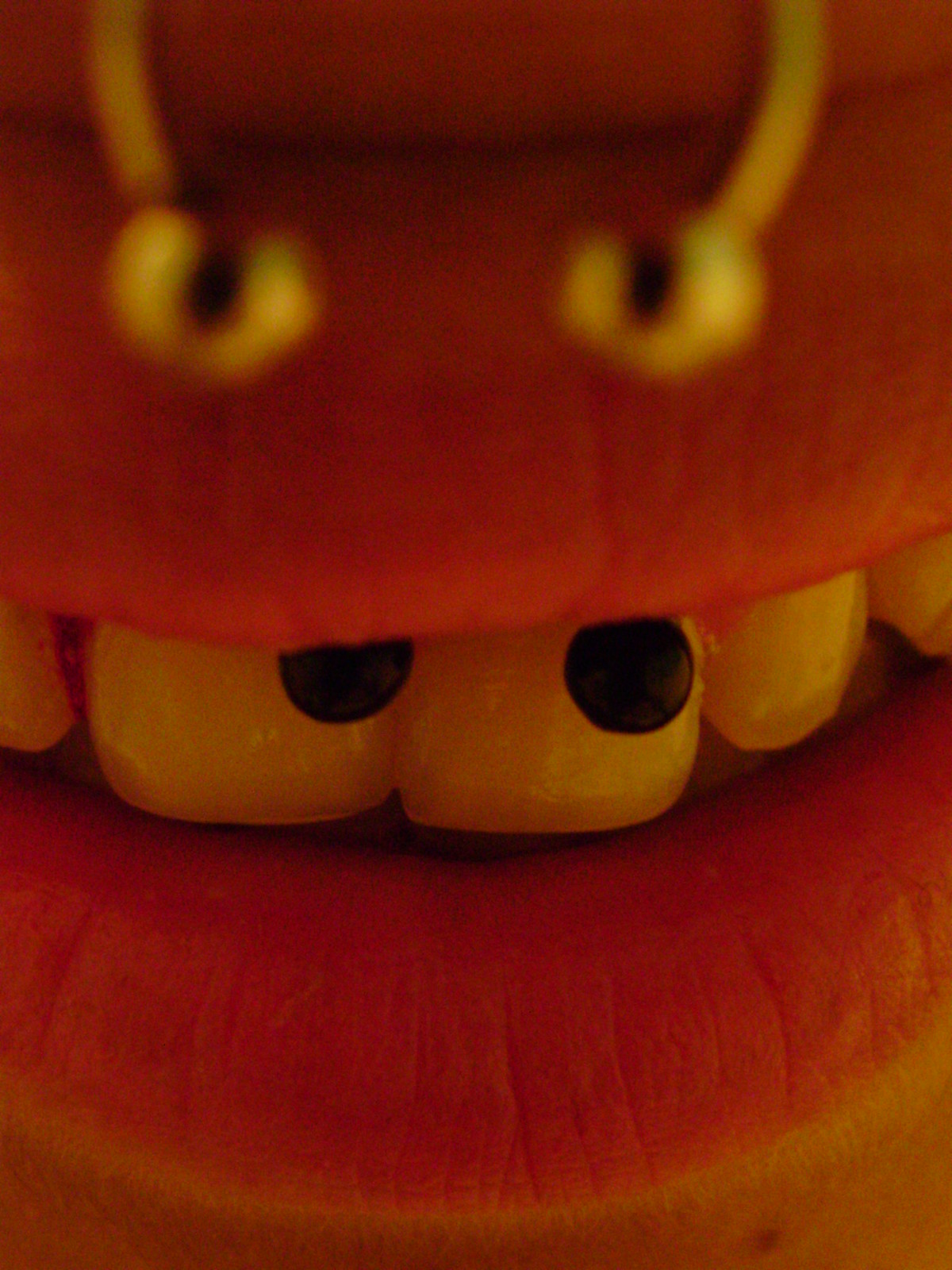This close-up image features a painted representation of a face on a person's mouth. The top lip is creatively adorned with two painted eyes, complete with upward-sticking eyelashes. Two black dots on the teeth mimic the nose of the imagined creature. The person's naturally pink lips, enhanced by lipstick, are prominently displayed, as is their light skin. A silver bull ring nose piercing with two balls at the tips hangs down adjacent to the top lip, and beneath the bottom lip, a piercing is visible, with its small balls resting near the teeth. Five teeth are clearly shown—two front teeth, the two on either side, and one adjacent tooth. The person’s tongue peeks slightly through the parted lips, and a freckle dots the chin just below the bottom lip. The composition tightly frames the mouth, excluding the full width of the lips and focusing only on the area immediately above and below them.